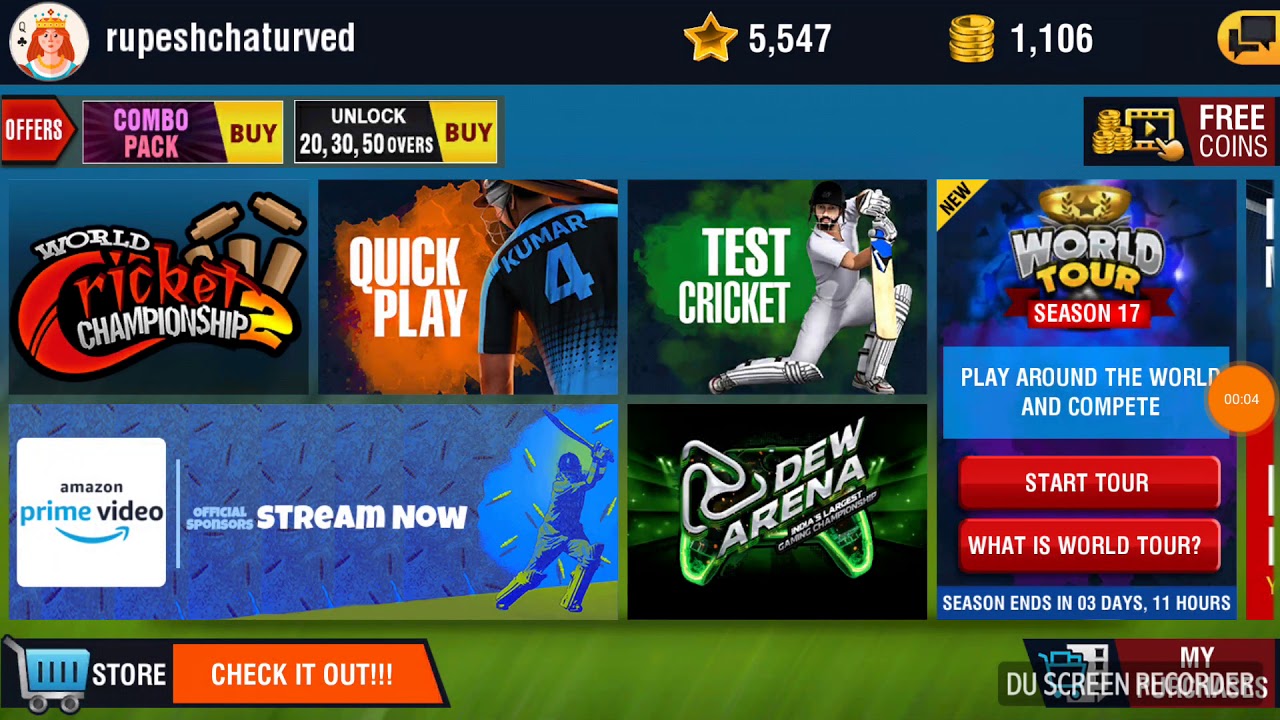This is a vibrant and colorful screenshot of a gaming website, showcasing a multitude of features and offers. At the very top, there's a black banner, prominently displaying a small profile picture of a cartoon princess with red hair, labeled "Rupees Shattered." Adjacent to the profile, there's a star indicating a total of $5,547 and a stack of cartoon coins valued at $1,106.

Beneath this section, a red banner titled "Offers" is visible, accompanied by multiple buttons for various actions: a combo pack purchase button, a button to unlock different tiers (20, 30, 50), another purchase button, and a button to earn free coins.

Below the banner, larger promotional offers are presented. One offer, titled "World Cricket Championship," features a blend of red, orange, yellow, and brown colors. Next, a "Quick Play" option is depicted alongside an illustration of a man with "Kumar" written on his shirt. Following this is an offer for "Test Cricket," showing an image of a man playing cricket.

An advertisement for Amazon Prime Video, labeling them as official sponsors with the phrase "In Stream Now," is also present. To the right, there's information about "World Tour Season 17," encouraging players to "Play Around the World and Complete." This section includes two red "Start Tour" buttons, an explanatory "What is World Tour" button, and a small orange button indicating a four-second countdown.